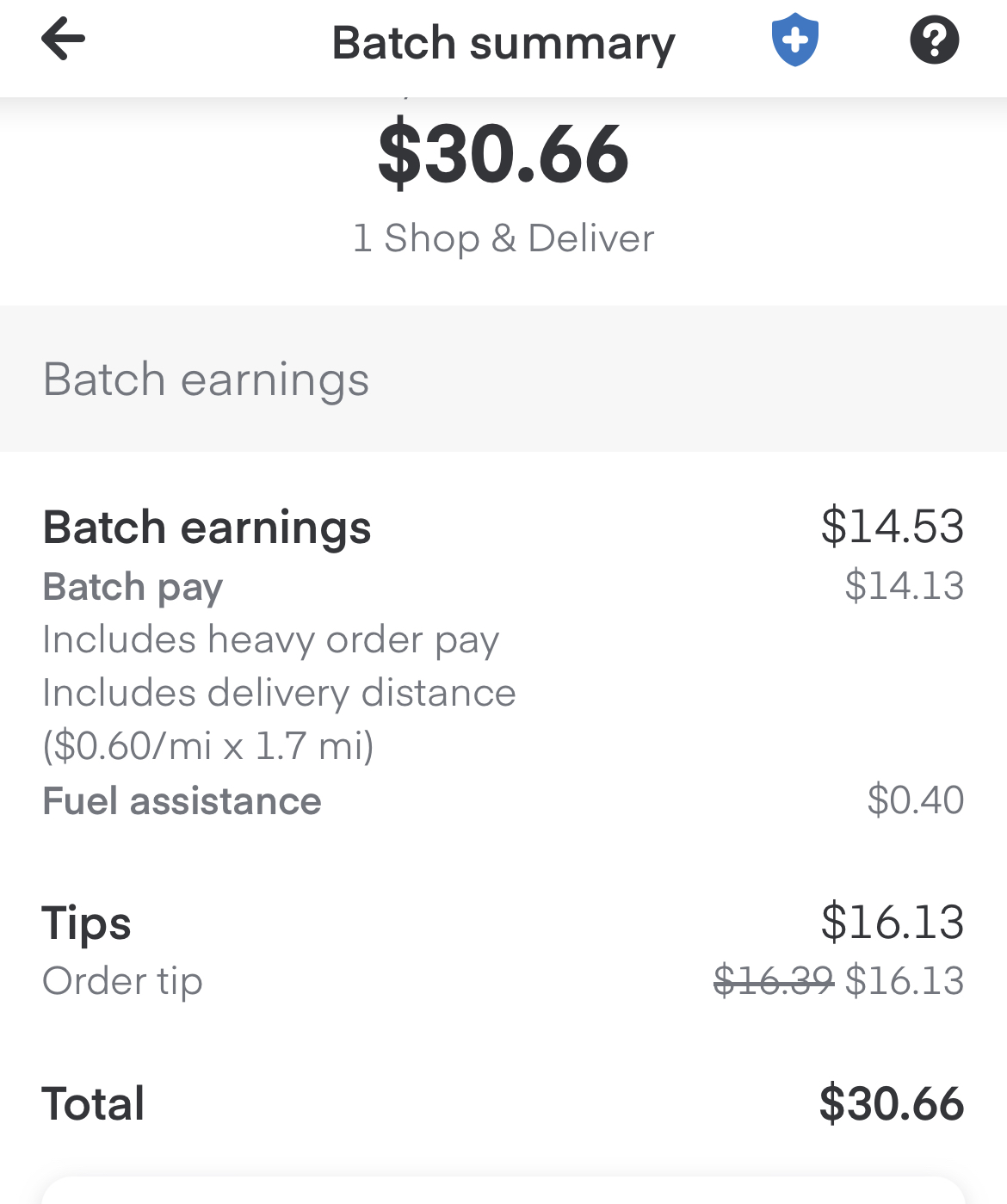**Batch Summary for One Shop and Deliver Order**

The webpage features a clean, structured design with a predominant white background. At the top, the heading "Batch Summary" is displayed in bold against a white backdrop, accompanied by an arrow pointing left and a blue shield with a white cross symbol.

Below, a black circle with a white question mark icon is prominently visible. Adjacent to this icon, the amount "$30.66" is displayed in large, bold black letters. Directly beneath this, in smaller gray text, it reads "One Shop and Deliver."

A gray box below this section is labeled "Batch Earnings." Inside this box, the text is detailed and organized as follows:

- **Header:** "Batch Earnings" in large, bold letters.
- **Earnings Breakdown:**
  - Batch Earnings: $14.53
  - Batch Pay: $14.13
  - Includes heavy order pay
  - Includes delivery distance: $0.60 per mile for 1.7 miles
  - Fuel assistance: $0.40
- **Tips:** Listed separately in bold black text as "$16.13"

The total earnings for the batch are reiterated at the bottom of the section: 
- **Total:** "$30.66" displayed in bold text.

Additionally, the order's tip amount shows an original figure of $16.39 which is crossed out and adjusted to $16.13, indicating a modification.

Overall, the webpage serves as a detailed receipt summary illustrating each component of the batch's earnings and adjustments in a straightforward manner.